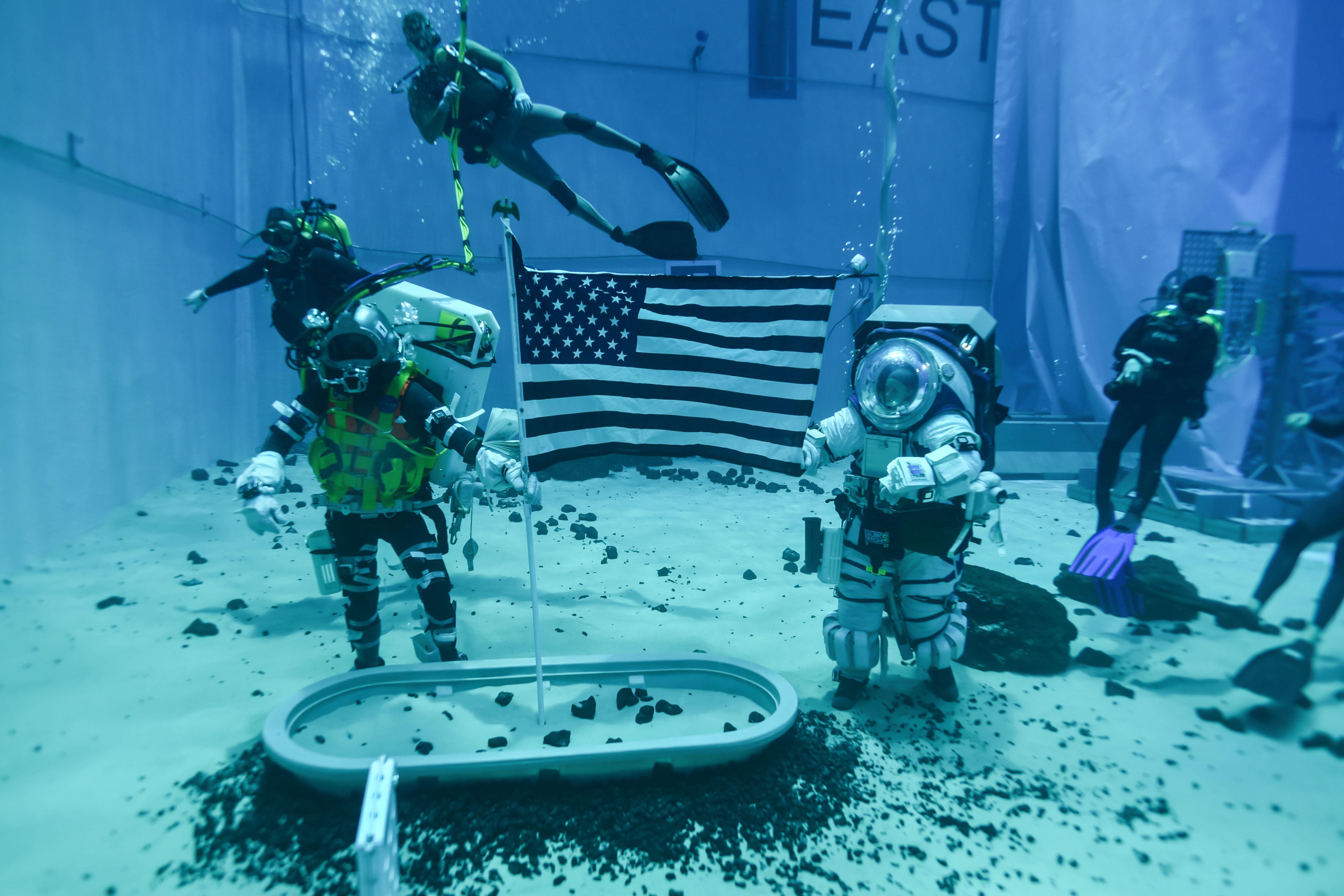The image depicts an underwater scene at the bottom of a deep blue-walled pool. Positioned centrally is an upright American flag embedded into a sandy bed. The scene features six individuals, five of whom are adorned in typical scuba diving gear consisting of black wetsuits, oxygen tanks, and flippers (with one diver sporting blue flippers). Notably, the sixth person is dressed in an astronaut's white space suit, complete with a large, clear globe helmet and a space backpack, mimicking a scene of weightlessness. The astronaut is positioned to the right of the flag, raising their arms. To the left of the flag, one of the divers has yellow straps securing their scuba gear. Film or research equipment is present, suggesting an orchestrated recreation, possibly for a movie or training. The word "east" is visible on the back wall of the pool. Overall, the image captures a fascinating juxtaposition of space and underwater exploration.